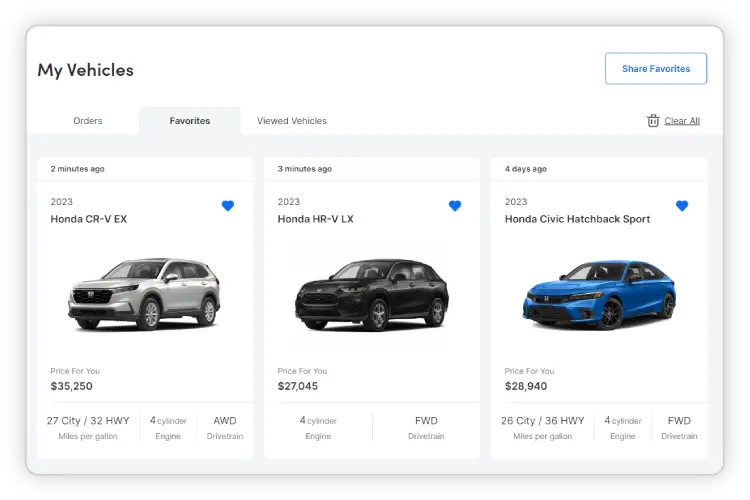This image is a detailed screenshot from a car dealership website or a vehicle management platform, showcasing a user interface that allows individuals to manage their vehicle interactions. The interface features a clean, white background, with the text "My Vehicles" prominently displayed in bold black font at the top left corner. On the far right, there is a white button outlined in blue with the text "Share Favorites" written in blue.

The user interface boasts a sleek and modern design. The toolbar seamlessly blends into the white background, with tabs highlighted subtly in gray to indicate selections. The toolbar's left side displays the tab "Orders" in gray text against the white background. Centrally located, the "Favorites" tab is highlighted with bold gray text on a softer gray background, showing it is currently in use. On the right side, the "Viewed Vehicles" tab is in gray text on a white background. Further to the right, there is a small gray trash can icon accompanied by the underlined text "Clear All."

As the "Favorites" tab is selected, the screenshot shows three favorited Honda vehicles. Each vehicle listing provides comprehensive details: 
1. A Honda CR-V EX, 2023 model, favorited two minutes ago.
2. A Honda HR-V LX, 2023 model, favorited three minutes ago.
3. A Honda Civic Hatchback Sport, 2023 model, favorited four days ago.

Beneath each vehicle listing, details such as the price, miles per gallon (MPG), engine specifications, and drivetrain information are clearly visible, providing a complete snapshot of the user’s selected vehicles.